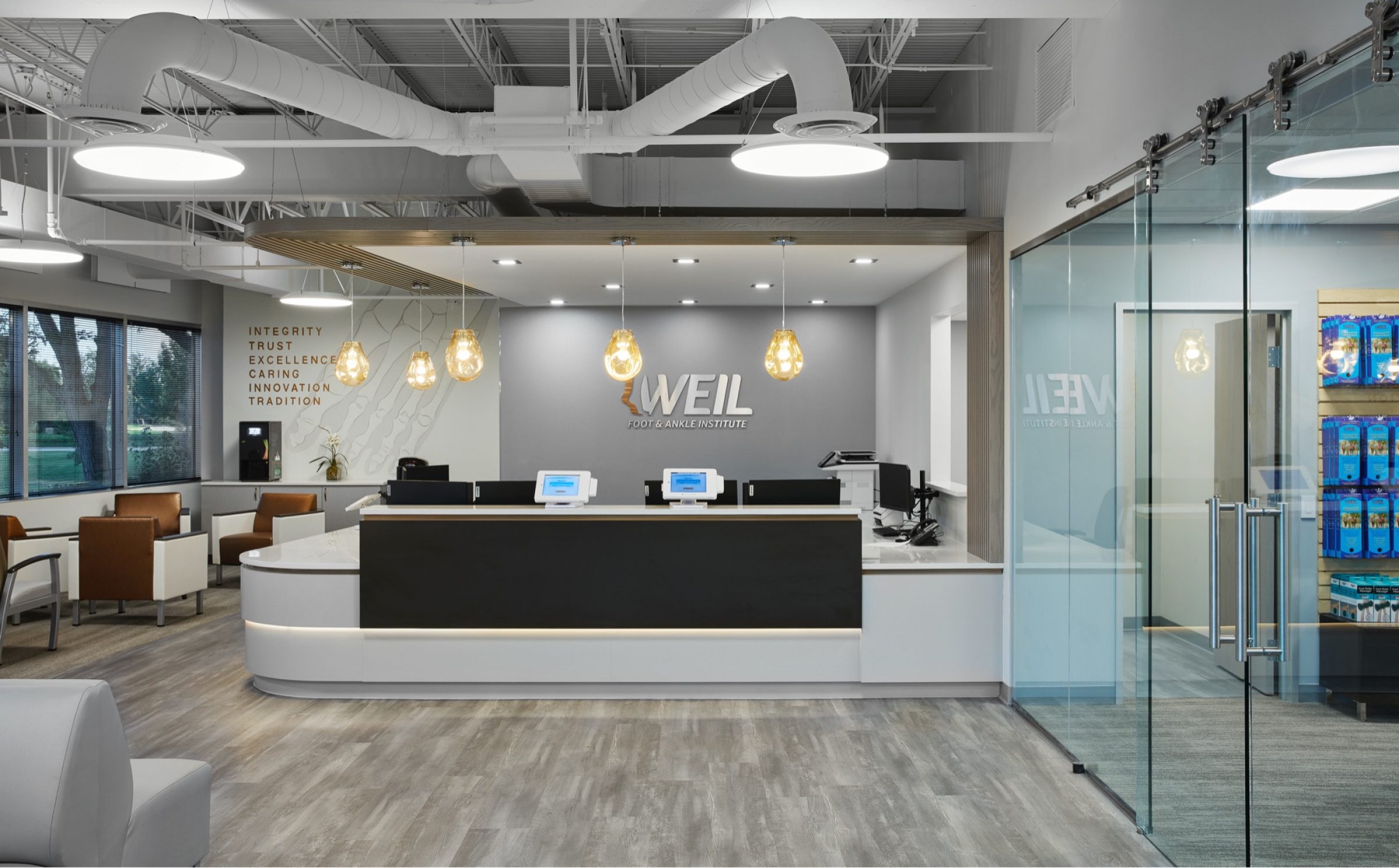The image showcases a modern office interior, potentially a 3D render, featuring an industrial yet clean aesthetic. The ceiling is exposed, revealing vents and pipes that are neatly arranged and painted gray and white, enhancing the contemporary look. Dominating the back wall is a gray surface adorned with the large, silver text "WEIL," accompanied by a smaller, unreadable text and a logo.

Suspended above the central office area is a unique lower ceiling section, characterized by wooden accents with white elements, which houses several inlaid circular lights. Adding to the intricate lighting design, metal fixtures with yellow bulbs hang from this structure.

The central area is enclosed by a desk, possibly where a receptionist or service personnel might be stationed, equipped with what appear to be tablets. On the left wall, the words "Integrity, Trust, Excellence, Caring, Innovation, Tradition" are prominently displayed. Below this text is a machine that resembles a coffee maker, adjacent to a seating area. 

The floor is covered in ash-gray, light wooden flooring laid vertically, contributing to the cohesive modern design. On the right side, glass doors open to another room, where a display wall showcasing blue products can be seen.